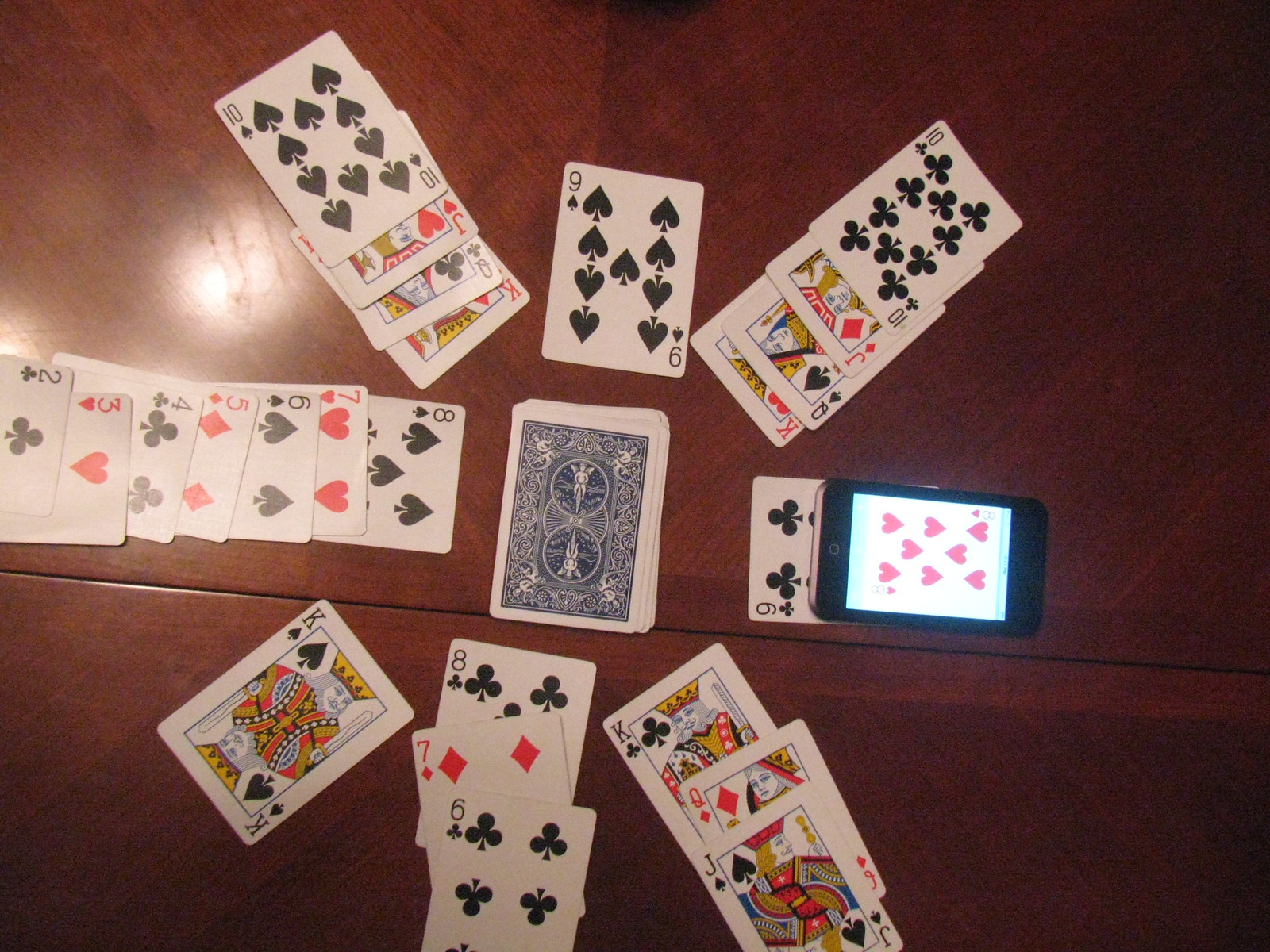In this top-down image of a game of cards, the scene is set on a wooden countertop or center table. The focal point of the image is a stack of playing cards in the center, with the top card being the 9 of spades. On the left side of the table, a sequence of cards is neatly aligned in a vertical line, consisting of the 8 of spades, 7 of hearts, 6 of spades, 5 of diamonds, 4 of clubs, 3 of hearts, and 2 of clubs.

On the right side, a 9 of clubs is prominently placed. Directly on top of this card lies an upside-down iPhone, which displays an image of the 8 of hearts on its screen. At the bottom of the image, a small cluster of cards includes the 8 of hearts, 7 of diamonds, and 6 of clubs.

Diagonally to the southwest, another grouping of cards features the king of diamonds, queen of clubs, jack of hearts, and 7 of spades in succession. Opposite this, on the northeast side, there is another set showcased with the king of hearts, queen of spades, jack of diamonds, and 7 of clubs.

In the bottom-right corner, a final arrangement includes the king of clubs, jack of diamonds, and jack of spades. The overall composition captures the organized chaos of a card game in progress, with strategic card placements and a glimpse of technology blending into the traditional game setup.